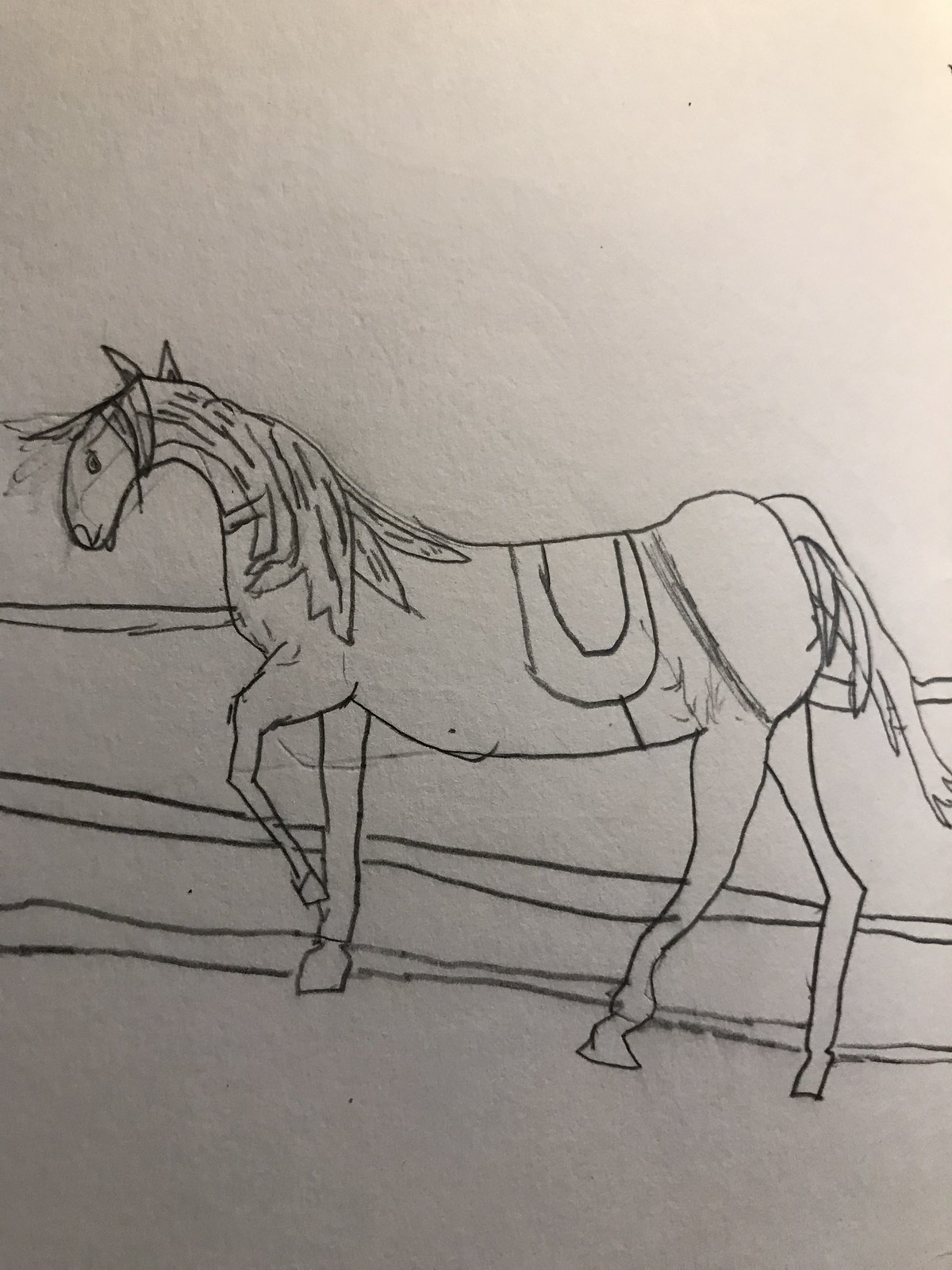In this minimalist drawing, likely created using a pencil, charcoal pencil, or ink, a horse is depicted in a side profile against a light gray backdrop. The rendering is straightforward, utilizing just a few clean lines with no shading. The horse, facing left, is adorned with a simplistic saddle represented by two lines. To the right, the horse stands beside a rudimentary fence, denoted by three horizontal lines. This artwork captures the essence of its subject with minimalistic elegance.